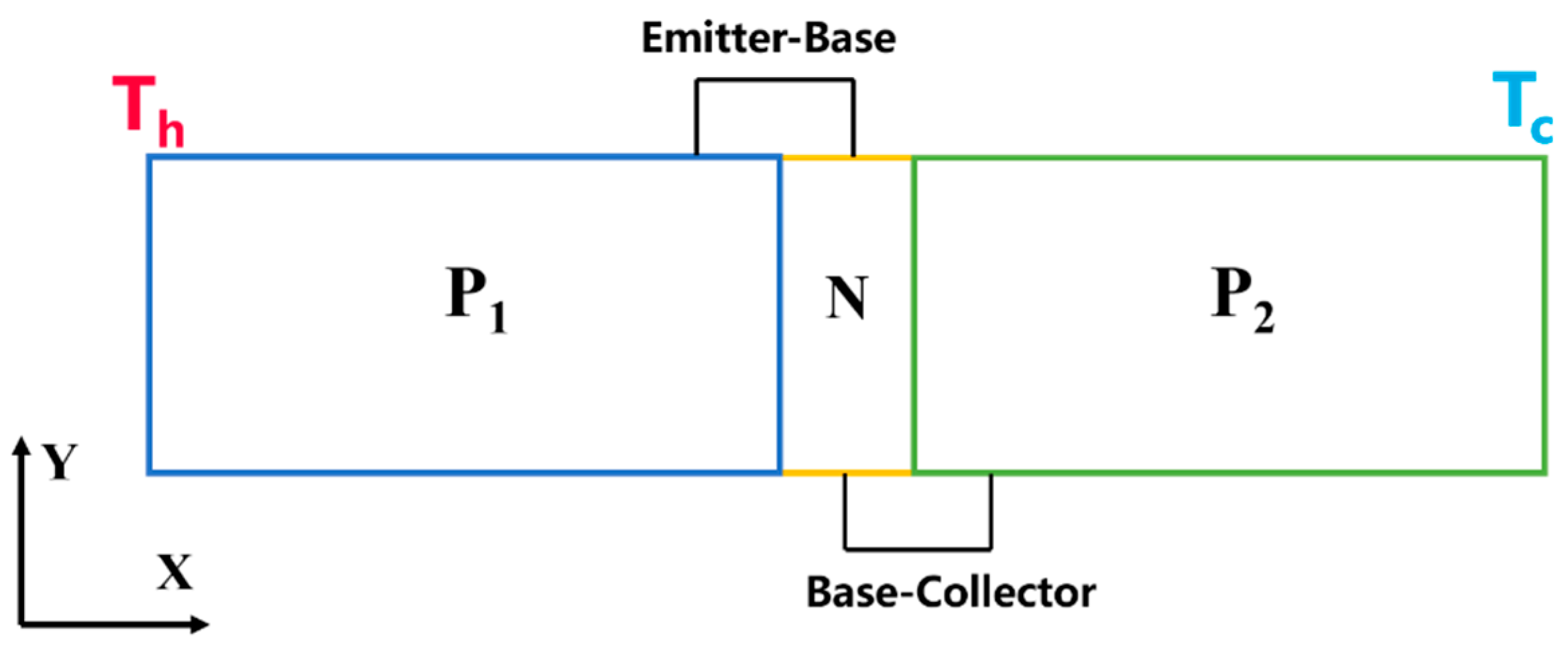The image is a detailed diagram on a plain white background, measuring approximately 6 inches wide and 2.5 inches high. The main elements consist of rectangular areas and connecting lines. 

On the left side, there's a blue-outlined rectangle labeled "P1" with "TH" in red font at its top left corner. In the middle, there's a vertically oriented section labeled "N" with yellow sides, connecting "P1" to another rectangle. On the right, another rectangle appears with a green outline labeled "P2," featuring "TC" in blue at its top right corner.

Above these components, there's a smaller rectangle labeled "Emitter Base" which connects the top of "P1" and "N" through a black line. Below, another small rectangle labeled "Base Collector" connects the bottom of "N" to the bottom of "P2" with a similar black line.

In the lower-left corner of the diagram, a black Y-axis extends upwards and an X-axis extends to the right, connecting at a 90-degree angle.

The diagram provides a clear visual of an implied system involving "P1," "N," "P2," their respective thermal points "TH" and "TC", and their electrical connections indicated by the "Emitter Base" and "Base Collector."